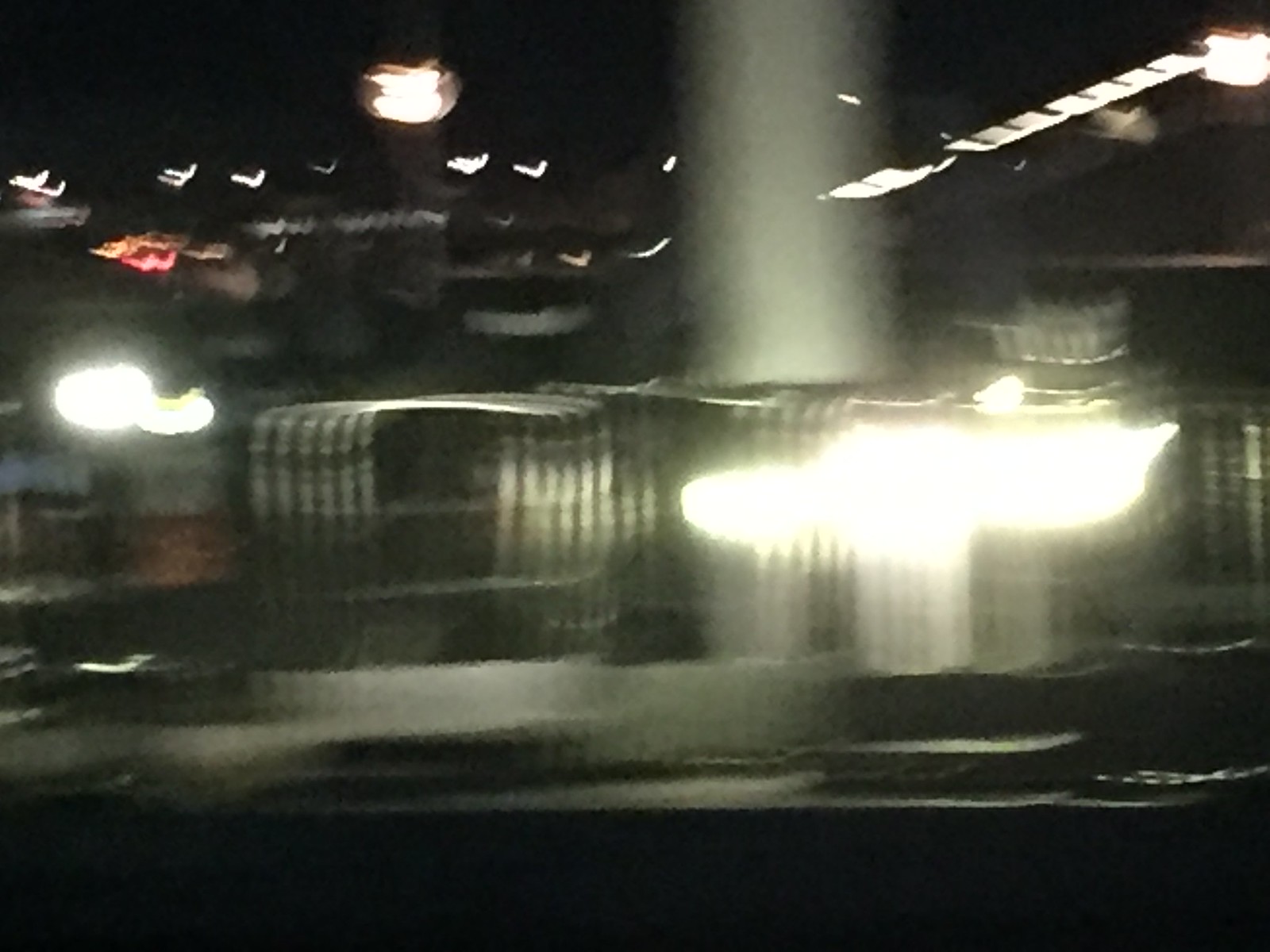A night-time colour photograph characterized by significant motion blur, making it challenging to discern specific details. The image captures a dark scene with a nearly black, thin line at the bottom that might indicate the edge of a structure or pavement. Above the line, there are several blurred lights, resembling a mix of fluorescent and smaller lights, scattered across the top of the frame. A larger light is positioned towards the left side, and a thick beam appears to descend near the center-right of the image, potentially indicating a structural element or post. There are vague, square-shaped outlines that suggest the presence of a gate or architectural feature. A particularly bright light near the center-right illuminates what seems to be platforms below. Additionally, a smaller bright light can be seen towards the center-left area of the photograph. The overall scene might depict a car park or the border of a building illuminated by various light sources in the dark, obscured by motion blur.